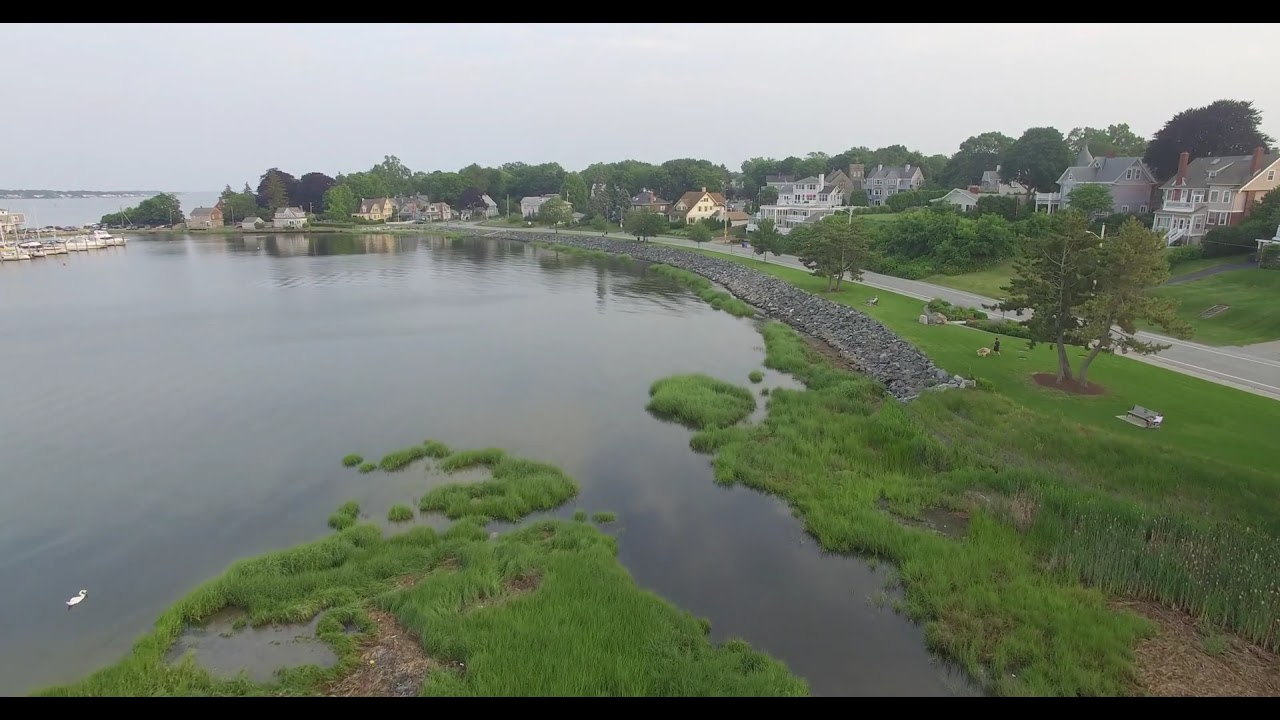The image portrays a picturesque aerial view of a serene waterside setting, featuring a small creek or pond embraced by lush green grass and tall trees. The creek winds through a charming residential neighborhood characterized by sizable two-story houses. Adjacent to the waterway, a lovely curved walking trail invites locals for leisurely strolls. On the left side, the scene transitions into a small harbour with white boats neatly docked, bordered by a bay that seamlessly integrates into the verdant landscape. 

Several people can be spotted enjoying the tranquility of the environment—some walking their dogs, while others sit contemplatively by the water’s edge. In the bottom left corner of the pond, a white swan gracefully glides through the water, adding to the idyllic nature of the scene. Across the waterway, more land extends into the distance, offering a continuous view of green space, rocks, and small patches of marshland. A few ventures and trees dot the grassy areas, enhancing the natural beauty of this refined neighborhood.